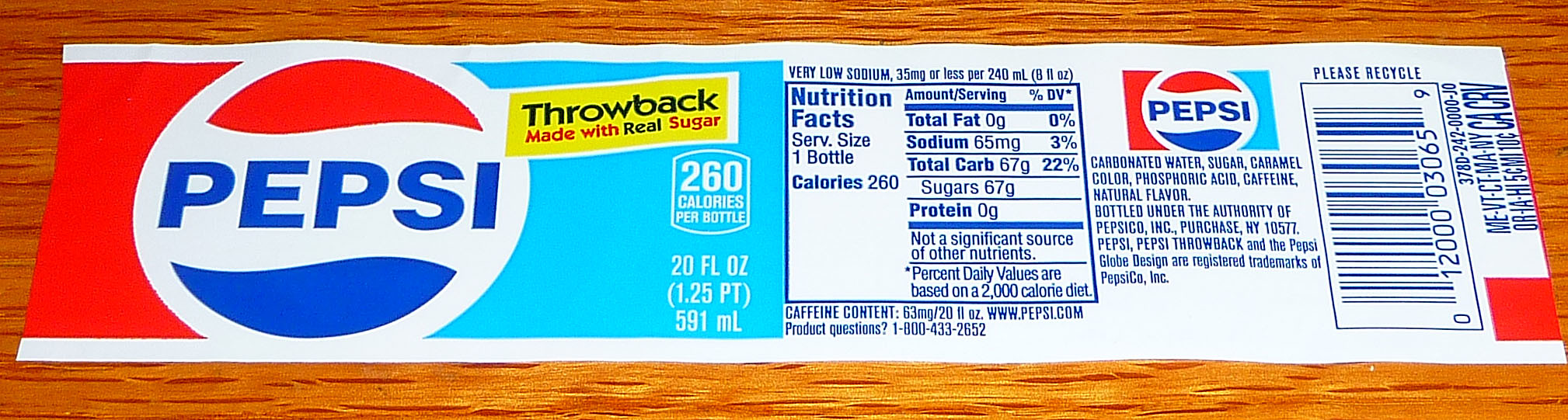This image features a peeled-off Pepsi label laying flat on a brown, wooden or laminate table. The label spans horizontally across the entire picture, with a small margin of the table visible on all four edges. 

The label starts with a red block of color, followed by the Pepsi logo—a white circle with a red swish on top, the word "Pepsi" in blue capital letters in the center, and a blue swish on the bottom. Next to the logo is a light blue area with a yellow banner that reads "Throwback, made with real sugar," where "Throwback" and "real" are in black, while "made with" and "sugar" are in red. 

Below this, in white text, it states "260 calories per bottle, 20 fluid ounces, 1.25 pints, 591 milliliters." The nutritional facts include serving size (one bottle), calories (250), very low sodium (35 milligrams or less), sodium (65 milligrams, 3% daily value), total carbohydrates (67 grams, 22% daily value), sugar (67 grams), and protein (0 grams). It mentions that it is not a significant source of other nutrients. Additionally, it notes that the percent daily values are based on a 2,000-calorie diet.

The caffeine content is listed as 63 milligrams per 20 ounces. The label also provides the website www.pepsi.com and a customer service phone number, 1-800-433-2852. Lastly, there is a smaller section with a smaller Pepsi logo, the ingredients (including carbonated water, sugar, caramel color, phosphoric acid, caffeine, and natural flavor), bottling information under PepsiCo Incorporated, New York, a barcode, and recycling information.